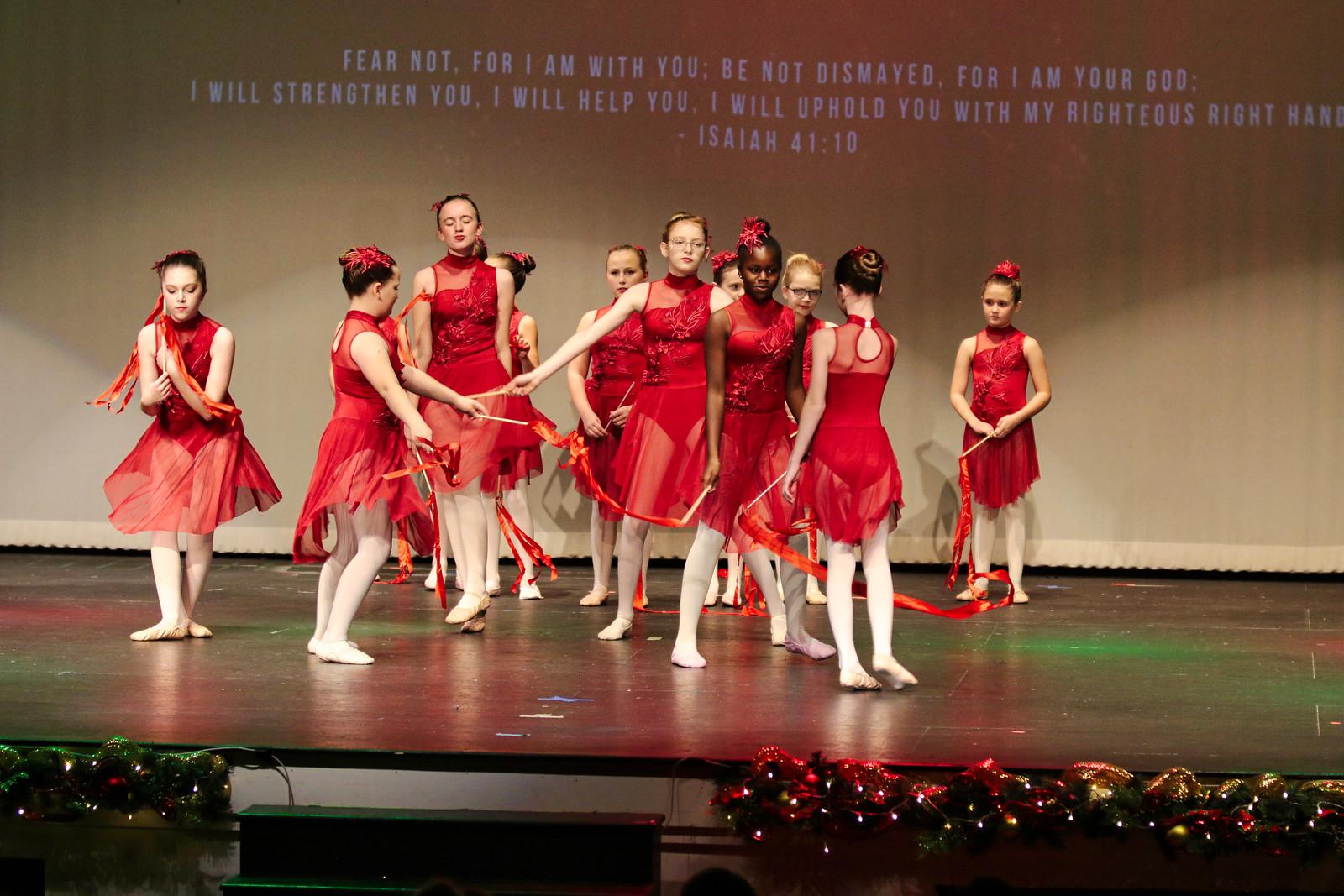This horizontal rectangular image captures a vibrant scene of a children's dance performance, likely themed around Christmas given the festive decorations. The stage is adorned with pine garlands intertwined with lights and tinsel, adding to the seasonal ambiance. In the middle of the image, a set of steps leads up to the stage, which is framed by a backdrop featuring a Bible verse from Isaiah 41:10: "Fear not, for I am with you. Be not dismayed, for I am your God. I will strengthen you. I will help you. I will uphold you with my righteous right hand."

On stage are twelve young girls, all dressed uniformly in sleeveless red dresses that extend to the neck and are paired with mesh skirts. Complementing their outfits, they wear white stockings and ballet shoes. Each girl has her hair pulled back, adorned with a red ribbon that coordinates with their costumes. Most of the girls hold white sticks, possibly as props for their dance routine.

The arrangement on stage features a cluster of girls in the center, some in motion, with two girls positioned at either end - one performing a dance step and the other standing still, holding an object. The overall scene showcases a meticulously coordinated performance, exuding both holiday cheer and a sense of spiritual encouragement from the scripted verse.